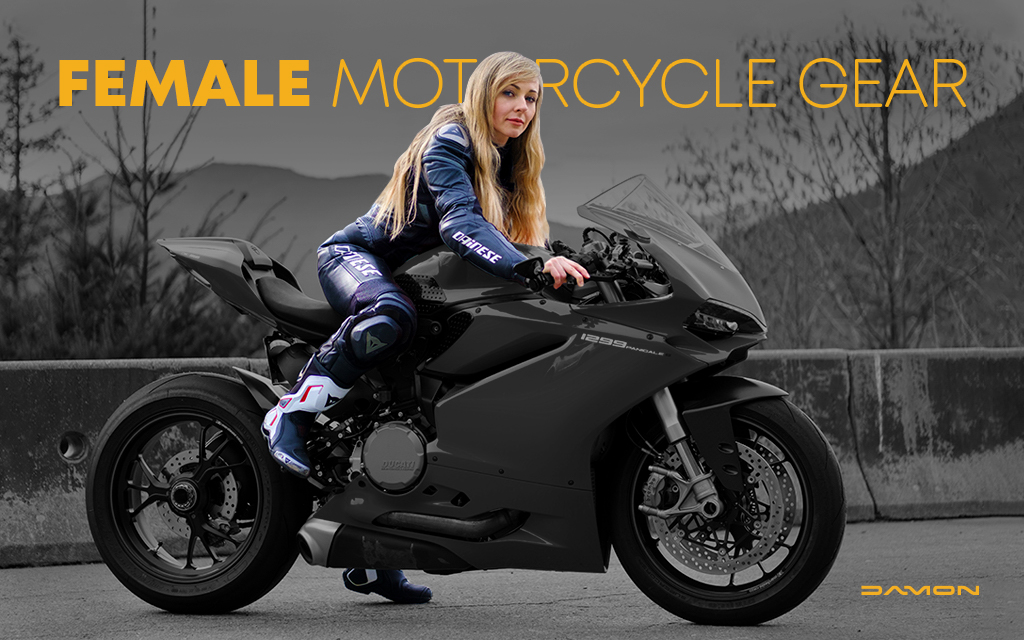In this grayscale advertisement for female motorcycle gear, a striking contrast is created by a vividly colorized woman riding a modern, curvy motorcycle along a road. Surrounded by a background of leafless trees, a gray mountainous landscape, and a worn-out concrete barrier, the picturesque outdoor setting emphasizes the boldness of the central figure. The woman, with her long blonde hair flowing almost to her waist, looks directly at the photographer. She dons dark blue motorcycle racing gear and holds the handlebars, her right leg poised on the bike and left leg on the ground, seemingly ready to start her journey. The advertisement features yellow text that boldly proclaims "Female Motorcycle Gear" across the image, with the brand name "Damon" stylishly embossed in the bottom right corner.